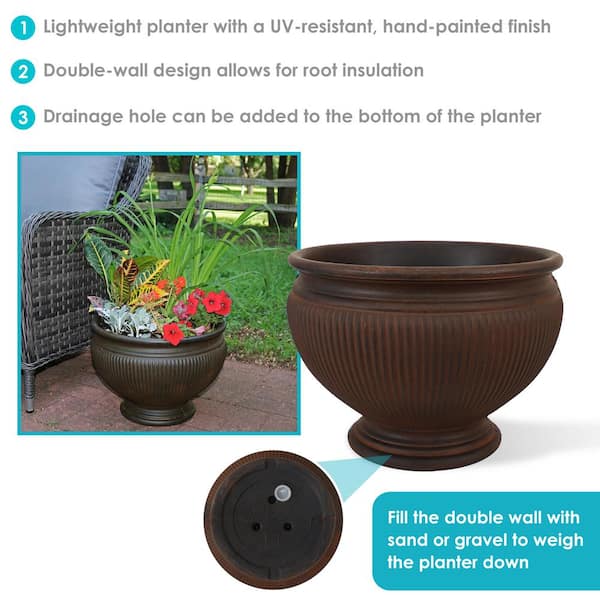This advertisement showcases an outdoor planter designed with both aesthetics and functionality in mind. At the top, clear instructions are numbered: 1) Lightweight planter with a UV-resistant hand-painted finish. 2) Double wall design allows for root insulation. 3) Drainage hole can be added to the bottom of the planter. The main image depicts the planter filled with vibrant red flowers and a mix of striking orange, yellow, and green foliage, placed on a brick patio beside a cushioned outdoor chair, with a backdrop that includes a grassy lawn, a split plank fence, and lush trees. To the right, a close-up of the empty planter highlights its detailed finish and another inset shows the bottom view, illustrating the potential for adding drainage holes. Beneath this, a blue text box with white writing instructs to fill the double wall with sand or gravel to weigh the planter down, ensuring stability.